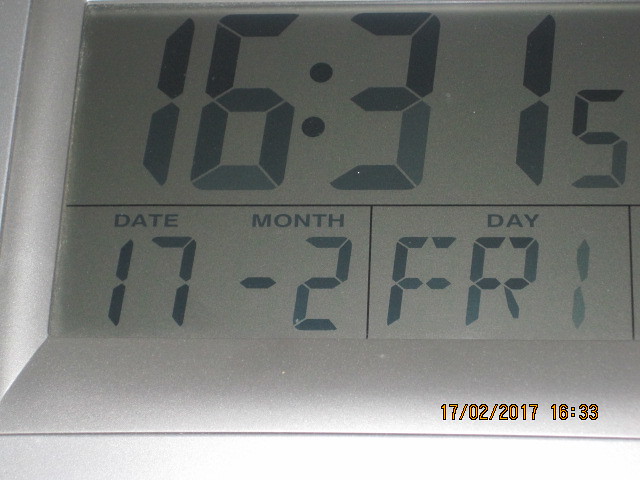A close-up image of a digital clock encased in a gray metallic plastic frame. The digital screen, with a plain gray-green background, shows the time as 16:31:50 (hours, minutes, and seconds). Additionally, the display indicates the date as "17-02" (February 17) and the day as "Friday." Despite the image being moderately illuminated with light entering from the bottom, the numbers appear somewhat faded, possibly due to the intensity of the light. A timestamp overlay confirms the date and provides a close time reading of 16:33 from February 17, 2017.